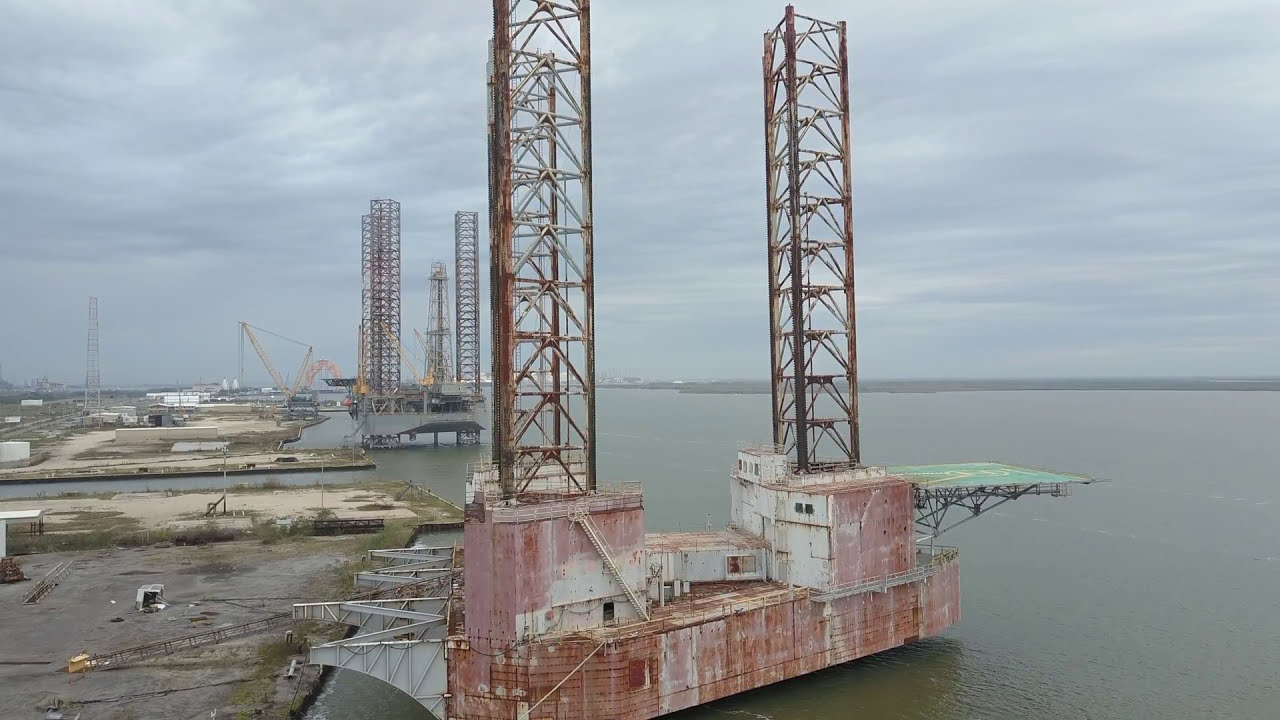This digital image captures an overcast, somewhat dreary view of a harbor, featuring several prominent and rusted oil derricks or rigs situated in brackish, brown water. The central focus is a heavily rusted, reddish-white barge with a green deck on its far right side, topped with two tall, rusty towers. In the foreground, there is a weathered helipad, which has faded from red to pink and white, situated on the right side of the barge. Another rig further in the distance is primarily gray and possesses similar towering structures. The surrounding land appears rugged and industrial, hosting various buildings and refineries. The photograph is taken from an elevated perspective, highlighting the juxtaposition of the decrepit, rusty rigs against the somewhat decrepit harbor backdrop. No text is present in the image, and it features a muted color palette including hues of red, pink, green, white, yellow, and blue, contributing to the overall sense of decay and abandonment.